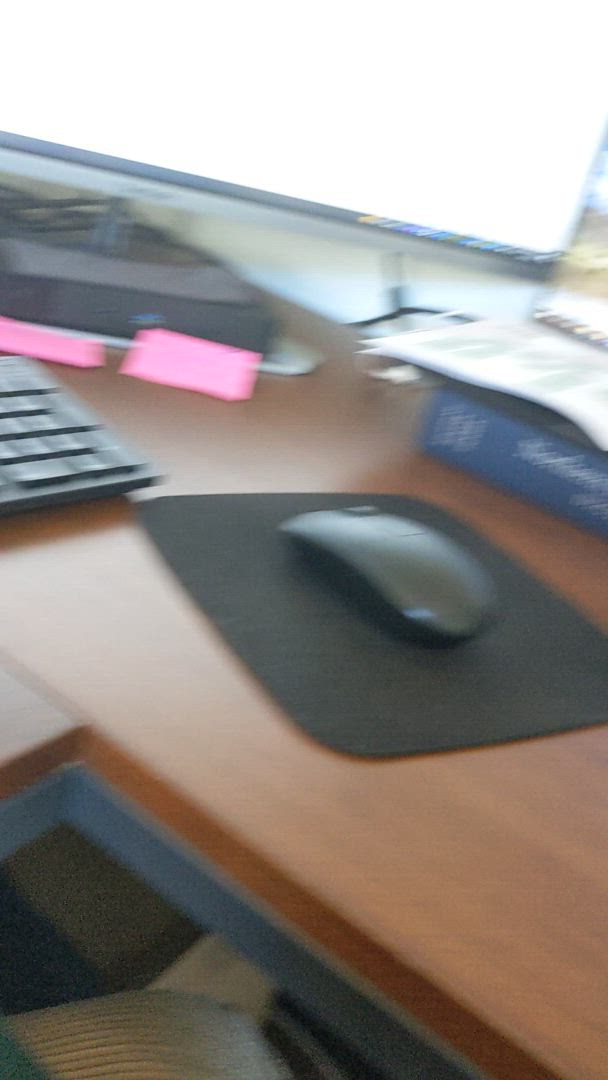A photograph captures the desktop of an office-style desk, although the image quality is marred by significant motion blur and is generally unclear. The surface of the desk is made of brown wood. Prominently displayed on the desk is a black rectangular mouse mat with a wireless mouse positioned on top of it. To the left of the mouse mat, there is a heavily blurred black keyboard. The base of a black monitor is visible in the background, while the bottom edge of the monitor’s screen appears to be white or grey. The monitor itself is overexposed, rendering the screen a bright white and obscuring any details.

In the background, a blue book with white writing on its spine lies on its side. The book seems to be around two inches thick. There is also some white paper extending out of the frame. Below the monitor, two pink post-it notes are visible, accompanied by a white cable running behind them. At the very bottom of the image, a section of white woven fabric is seen, which could either be part of a chair in front of the desk or the clothing of the person seated at the desk.